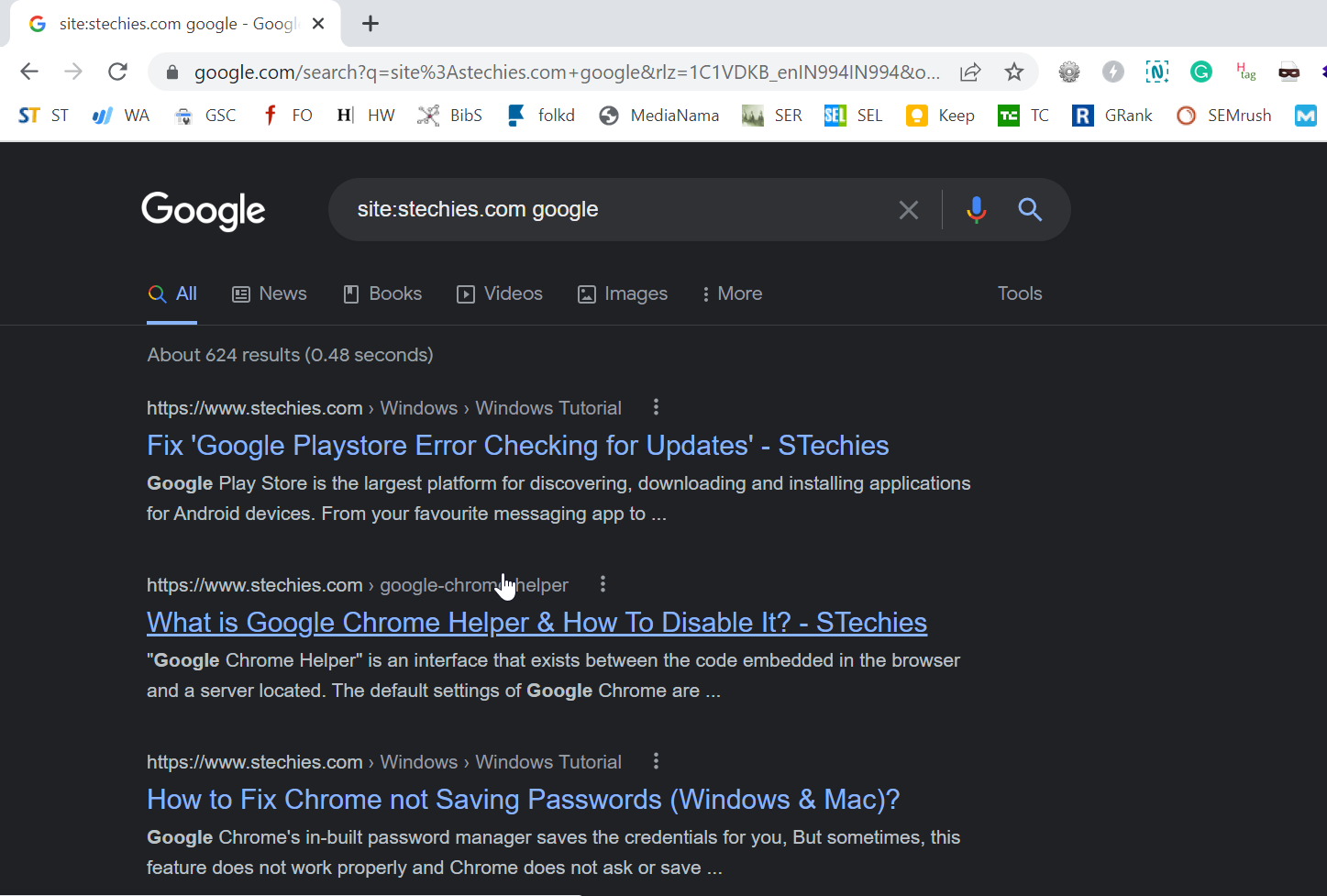This image is a detailed screenshot of a Google search results page, captured in dark mode. The background of the page is black, highlighted by contrasting text in white, light gray, and blue. At the top of the page, the URL bar displays "google.com/search" along with additional query parameters, and features a closed lock icon indicating a secure connection.

The browser's bookmark bar is visible, showcasing several bookmarked pages. Prominently placed towards the top-left of the page is the Google logo, rendered in white, adjacent to an active search bar containing the query "site:sketches.com google."

Below the search bar, several menu options are listed: "All," "News," "Books," "Videos," "Images," "More," and "Tools." Three search results are displayed within the screenshot. Each result consists of a URL, the title of the page highlighted in blue, and a brief descriptive snippet of text summarizing the page's content.